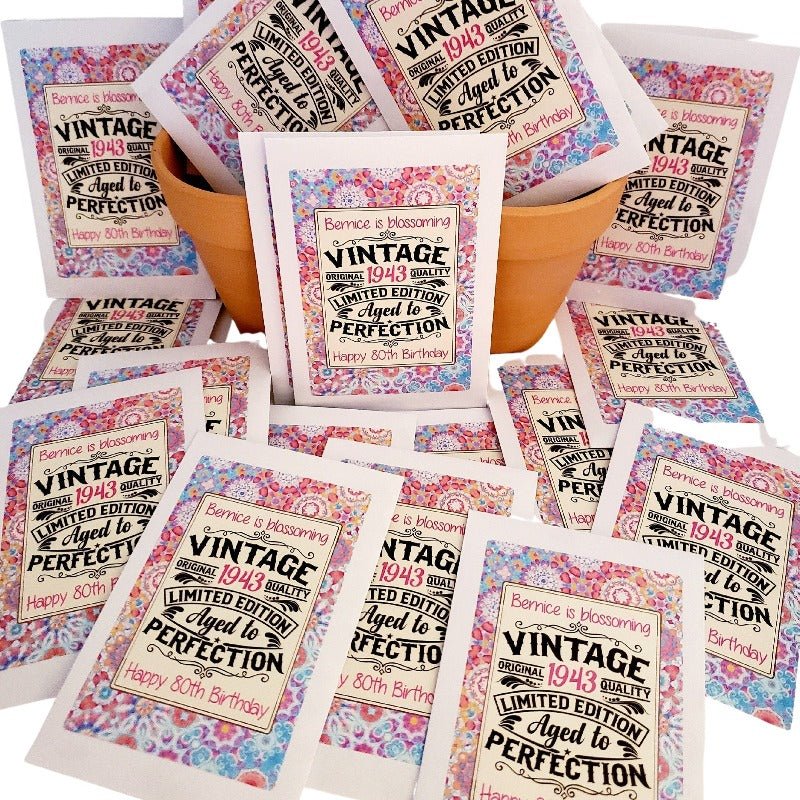The image appears to be an advertisement resembling a catalog display. It showcases multiple birthday cards, all with a playful vintage theme celebrating an 80th birthday. The cards, which bear celebratory messages such as "Bernice's Blossoming Vintage 1943, Limited Edition, Aged to Perfection. Happy 80th Birthday," are arranged around two orange clay flower pots situated in the upper center of the image. The cards feature a colorful floral pattern with red and blue hues around a white-bordered yellow rectangle, where the text is highlighted in black and the year "1943" is prominently displayed in red. The whole arrangement is set against a completely white background, with some cards neatly tucked inside the flower pots and others scattered around their base, creating a visually appealing composition.